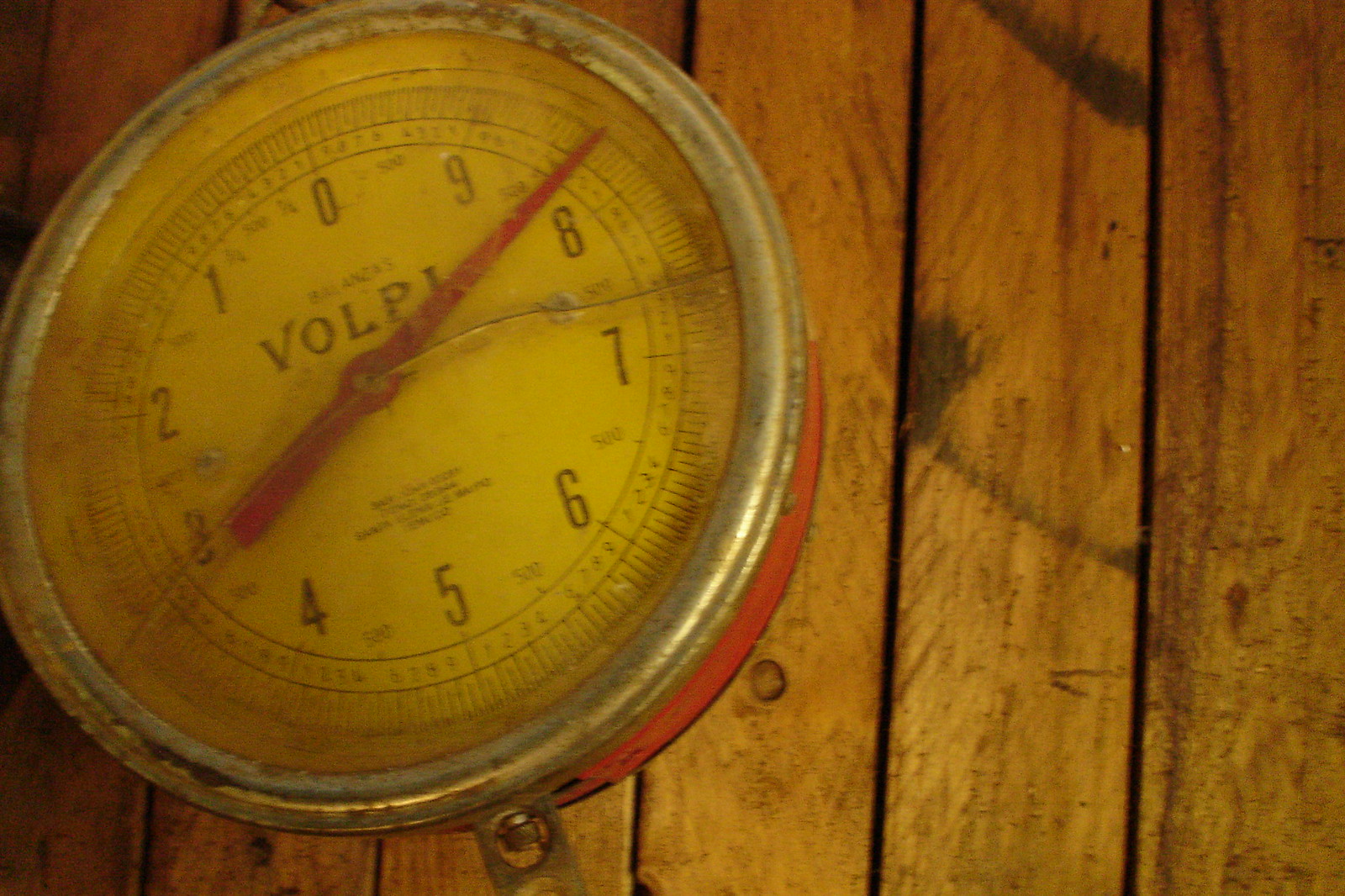A heavily damaged vintage Volpe weighing scale is resting on a wooden board. The scale appears to be in disrepair, with significant visible breakage.